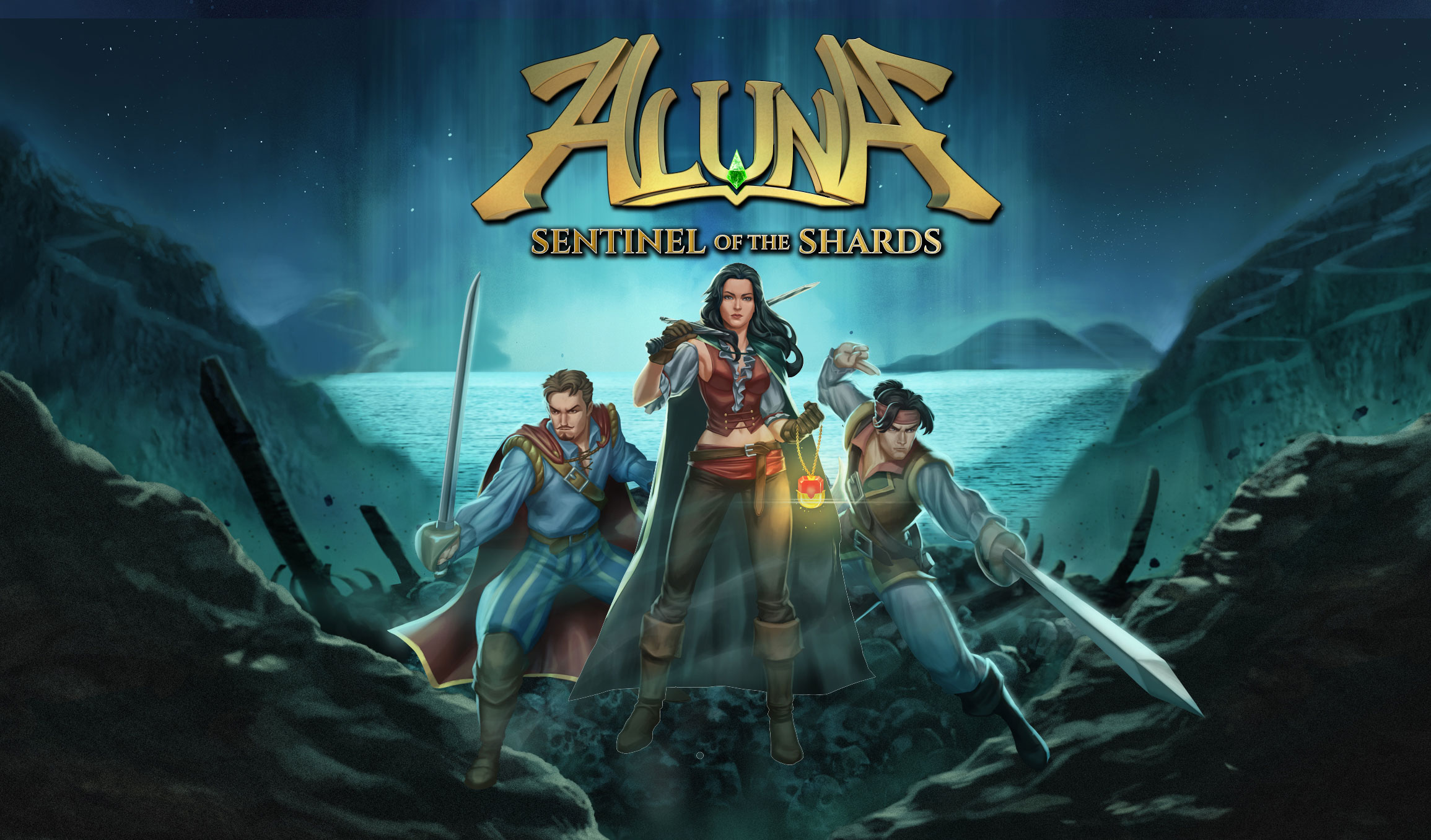This vibrant, rectangular advertisement, likely for a mobile game or an anime, features the title "Aluna: Sentinel of the Shards" prominently in golden letters at the top. The backdrop is a mystical landscape in deep blues, dark greens, and blacks. The foreground introduces three central characters ready for battle, framed against a dramatic scene with oceanic and mountainous elements. At the center stands a poised female warrior, distinguished by her long dark hair and dressed in a purple vest with knee-high boots, a sash, and leather pants, holding a sword over her shoulder. Her confident gaze is directed towards the viewer. Flanking her are two male companions, each brandishing a sword, dressed in blue, brown, and gray attire. The man to her left, adorned with a goatee and a large brown cape, seems braced for action, while the man to her right, distinguished by his bangs, stands equally ready. Together, they convey a sense of preparedness and unity amidst the dark, mystical setting.